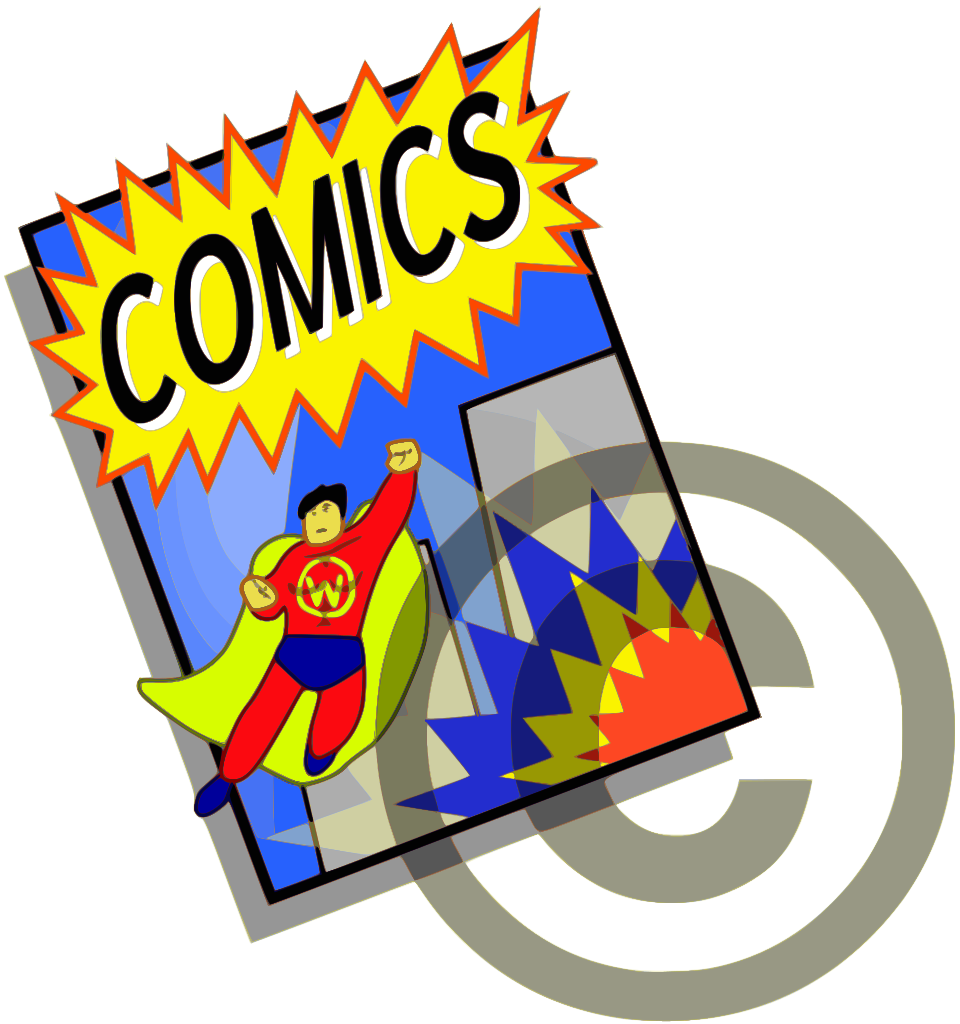The image is a digital clipart depiction of a comic book with a white background and a watermark, a giant "sea," overlaying the entire picture. The comic book image is positioned in the top left corner and leans diagonally to the left. The cover primarily features a blue background with a prominent yellow starburst outlined in orange, where the word "COMICS" is displayed in black capital letters with a white drop shadow. Within the comic book scene, a superhero with minimal facial details is featured in the bottom left corner. The character, reminiscent of Superman, has black hair, a yellow face, and wears a red shirt with a "W" emblem inside a yellow circle, red pants, and blue underwear-style tights. He also sports a neon yellow cape and blue shoes. The superhero strikes a classic pose with one fist raised as if flying. Two rectangles indicating tall skyscrapers are behind him. In the bottom right corner of the comic book, a series of explosive starburst illustrations in blue, yellow, and orange add dynamic elements, with each explosion progressively smaller than the one behind it. The colors in the image include orange, yellow, blue, black, white, gray, and lime green, contributing to the vibrant, dynamic style typical of comic book art.